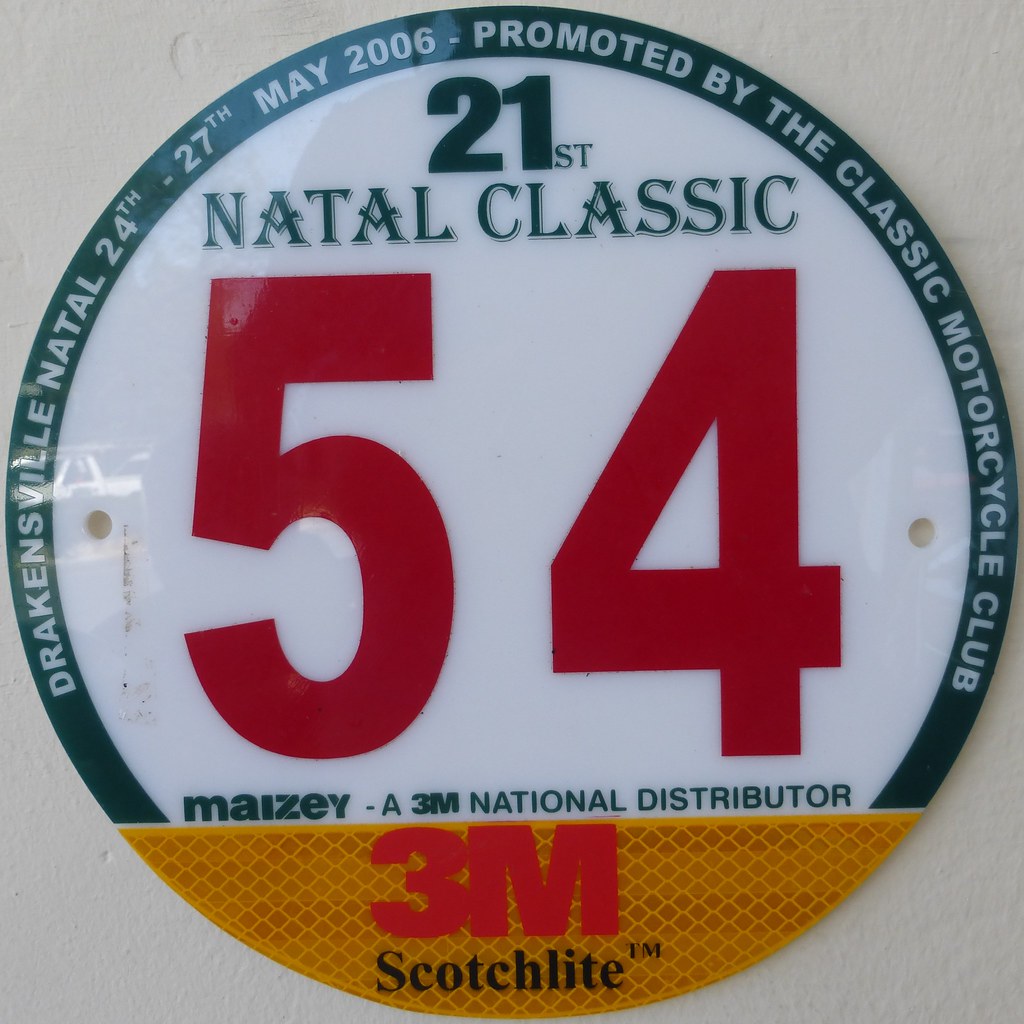This square photograph showcases a round sign mounted against a white stone wall. Encircling the sign is green and white text that reads: "Great Brazil Natal 24th-27th May 2006, promoted by the Class Motorcycle Club." Dominating the center of the sign are the large green letters "21st Natal Classic" with an oversized red number "54" prominently displayed below. Beneath this, in smaller green text, it states "MAIZEY-3M National Distributor." Across the lower portion of the sign, there's a yellow section imprinted with "3M Scotchlite." The sign is outlined in green, and the overall design suggests it's a commemorative piece or promotional artifact related to a motorcycle event.